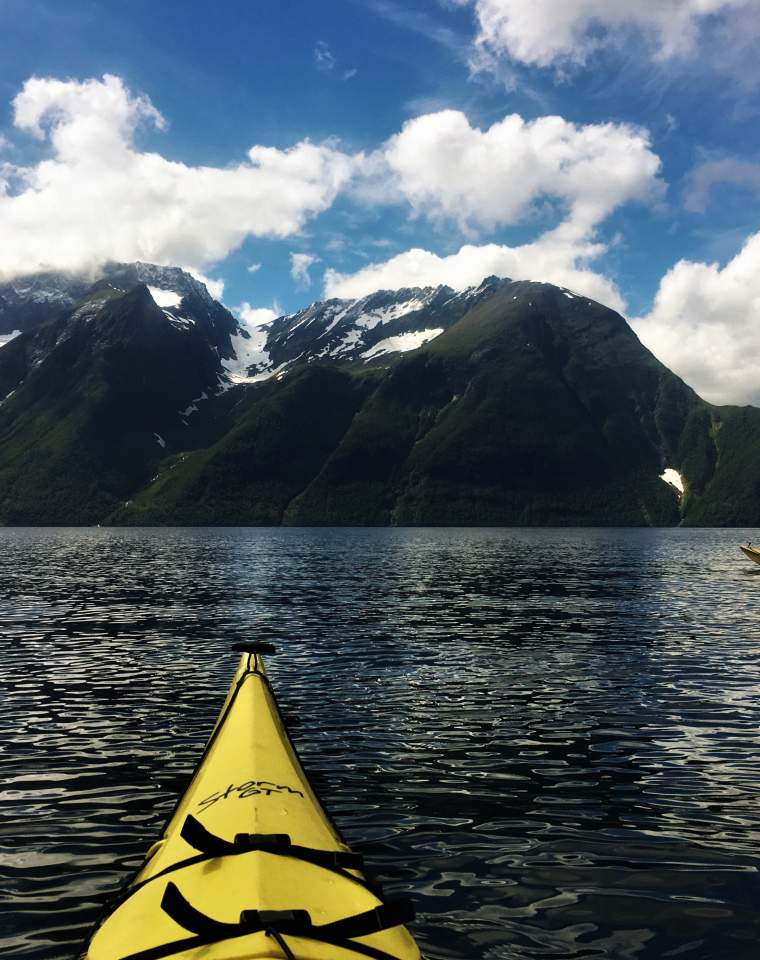In this vertical photo, the viewer's perspective comes from the front of a yellow kayak outfitted with black straps. The kayak is navigating a serene, slightly rippled body of water. The water's dark hue suggests a depth beneath its surface, gently disturbed by a light breeze. In the distance, a grand mountainous region rises dominantly from the water, its rugged cliffs adorned with patches of green moss and trees clinging to the steep slopes. The mountain's peaks are capped with glistening snow, adding a touch of contrast against the earthy tones of the cliffs. Above, the sky stretches out in a clear, deep blue, dotted with white clouds that seem to hug the mountain tops, particularly on the left side. The scene captures a tranquil yet awe-inspiring moment of natural beauty, as the adventurer in the kayak paddles onward.